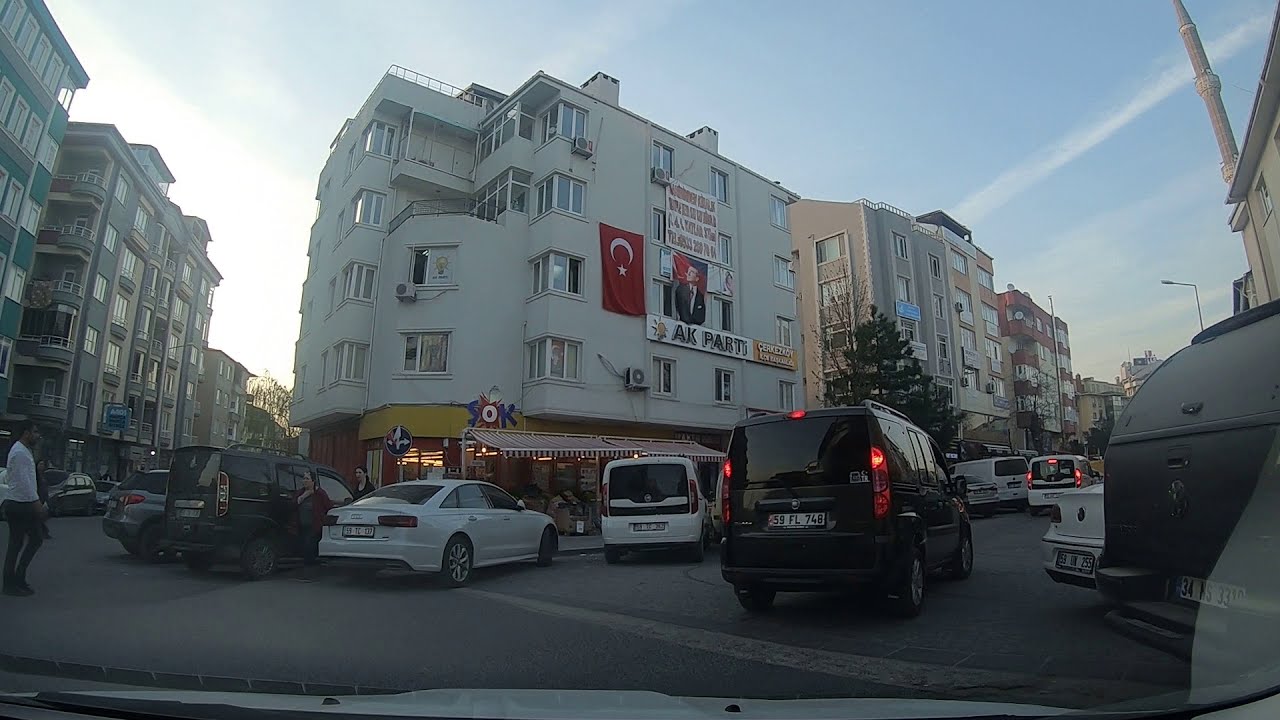The image captures a bustling urban street intersection viewed from the interior of a vehicle in the middle of a right turn. The road, constructed with dark gray bricks, is vibrant with activity. A black van, bearing the license plate 59FL748, is also turning right ahead. The backdrop features a deep blue sky with long white clouds and a partially setting sun on the left, illuminated by the soft glow of twilight.

Multiple parked vehicles line the street, especially noticeable in front of a large multi-story white stone building with distinct white and blue “S-O-K” lettering on a striped red and white awning below, indicating a business, likely a restaurant, at the street level. Above it rises four stories, possibly part of an apartment complex, adorned with a banner featuring a man's image and the inscription "AK Party."

Further down the street, additional apartment complexes in shades of light brown and dark brown are visible. On the left side of the image, beyond the busy road, there are more buildings in green and gray tones. A pedestrian dressed in black pants and a white long-sleeve shirt is seen walking towards one of the parked cars in front of the building, contributing to the lively atmosphere of this urban scene.